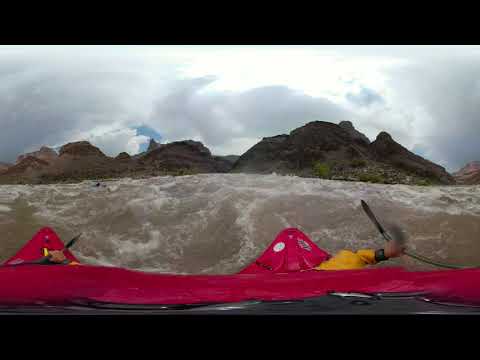In this 360-degree image, a turbulent and murky brown river with numerous white-capped waves navigates through a rugged canyon. A red kayak dominates the scene, with its rounded triangular front visible on the right side of the image and its back extending to the left. A person, visible only by their arms and hands, is struggling to control the kayak in the choppy water. The person is clad in yellow waterproof clothing, with black wrists, gripping a long black paddle on both sides of the kayak. The left hand is positioned lower, and the right hand holds it higher, but the right hand isn’t fully visible. Surrounding the river, the canyon walls rise steeply, consisting of high, jagged rocky hills and crags. Above, the sky is heavily clouded with a hint of sun brightness diffusing through the dense clouds, and a small patch of blue sky peeks out, adding contrast to the otherwise overcast scene.